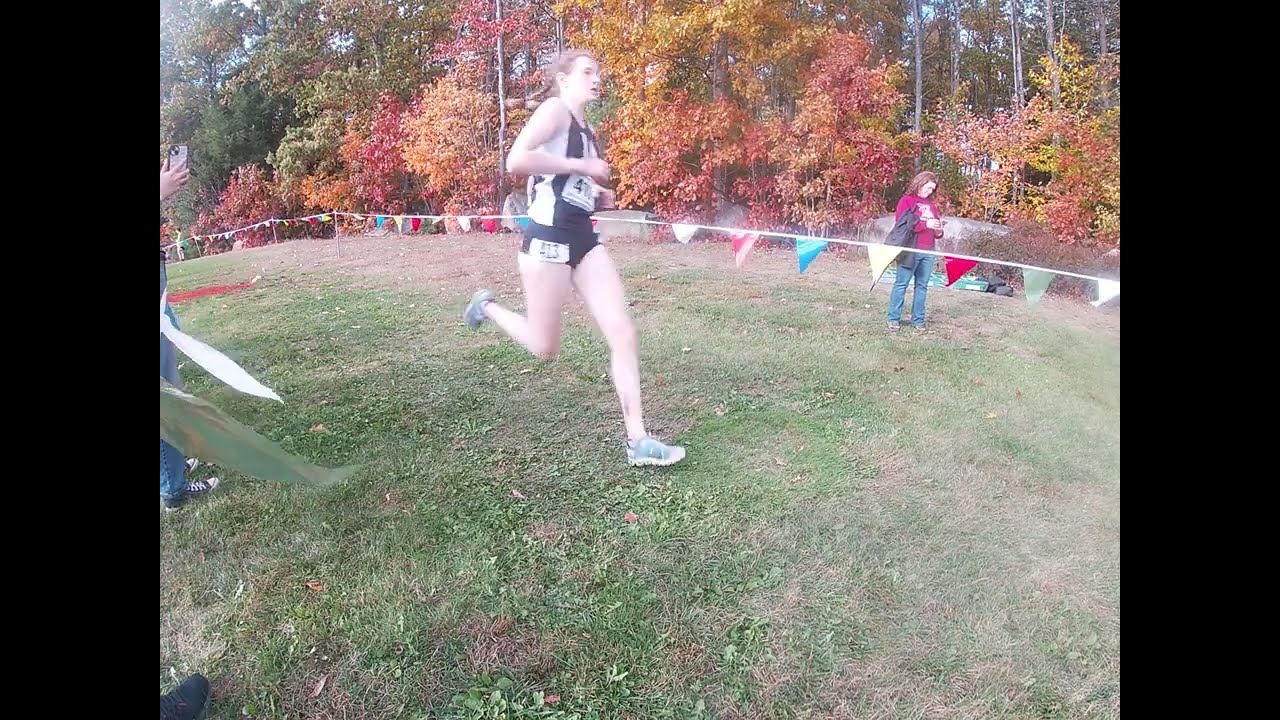This photograph, likely a screenshot from a video, captures a female track runner participating in a race and wearing number 413. She is dressed in black shorts and a black sleeveless tank top with a white stripe on the side, complemented by running shoes. The scene is set outdoors on a grassy terrain, which appears to be in the early stages of autumn, evidenced by the trees in the background showing a vibrant mix of reds, oranges, yellows, and some still-green foliage. Behind her, a long rope adorned with red, green, yellow, and blue triangular flags flutters in the wind, marking the boundary between the race area and spectators. To the right in the background, a person in a red top and blue jeans, with a coat draped over their arm, is engrossed in their phone. On the left, partially cut-off individuals are seen taking pictures or filming the event. The entire image is framed by black vertical bars on both sides, enhancing the focus on the runner who appears to be isolated, either leading or trailing in the race.